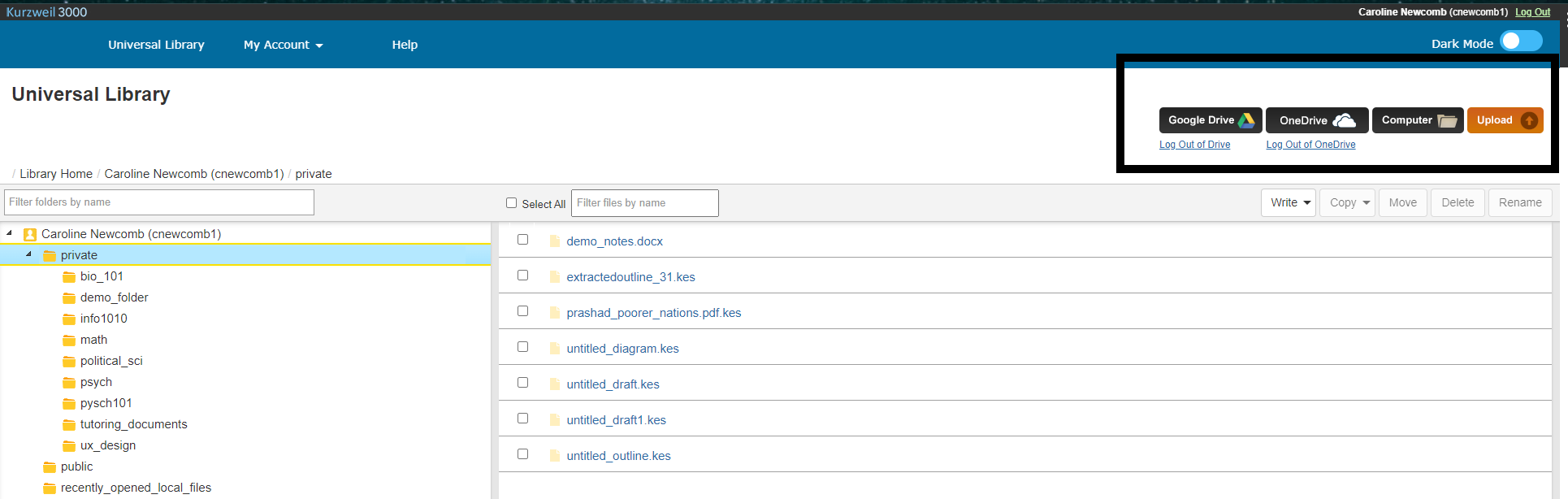This image is a detailed screenshot of a lookup interface within a platform called Universal Library. In the upper left corner, the title "Universal Library" is prominently displayed, with "Library Home" positioned just below it. The interface showcases several folders; some discernible names include "Political," "PSYCH," and "PSYCH 101." On the right side, additional folders are visible, though many of the names are blurred and difficult to read, with some beginning with "Untitled." At the top right corner, there is a black box highlighting various buttons with links, likely for navigation or uploading purposes. These buttons include "Google Drive," "OneDrive," "Computer," and possibly "Upload."